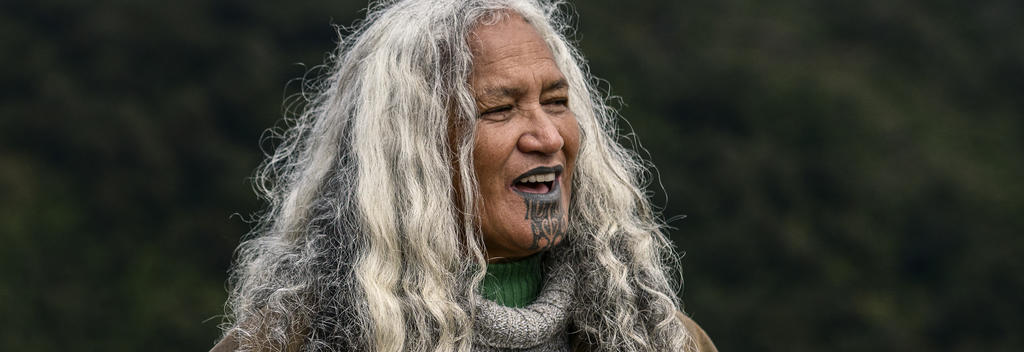The image captures an older individual, possibly a man, with long, curly, gray, and white hair. His hair appears frizzy but not tightly coiled. The person's medium-dark skin and facial tattoos — black lips with tribal patterns extending over the chin — suggest he may be of Maori or New Zealand indigenous descent, though this is not explicitly identified. He is dressed in layered clothing, with a green turtleneck sweater underneath a thicker, gray cowl-neck sweater. The background is an out-of-focus blend of green hues, indicating the photograph was taken outdoors and uses a shallow depth of field to accentuate the subject. The even sunlight creates a soft, natural light on his face, which looks composed and serene, possibly with a faint smile as he gazes into the distance. His facial features are distinctive, with puffy eyes, a broad nose, and high cheekbones, and the overall photograph is notably wide in format, spanning approximately three or four times its height.